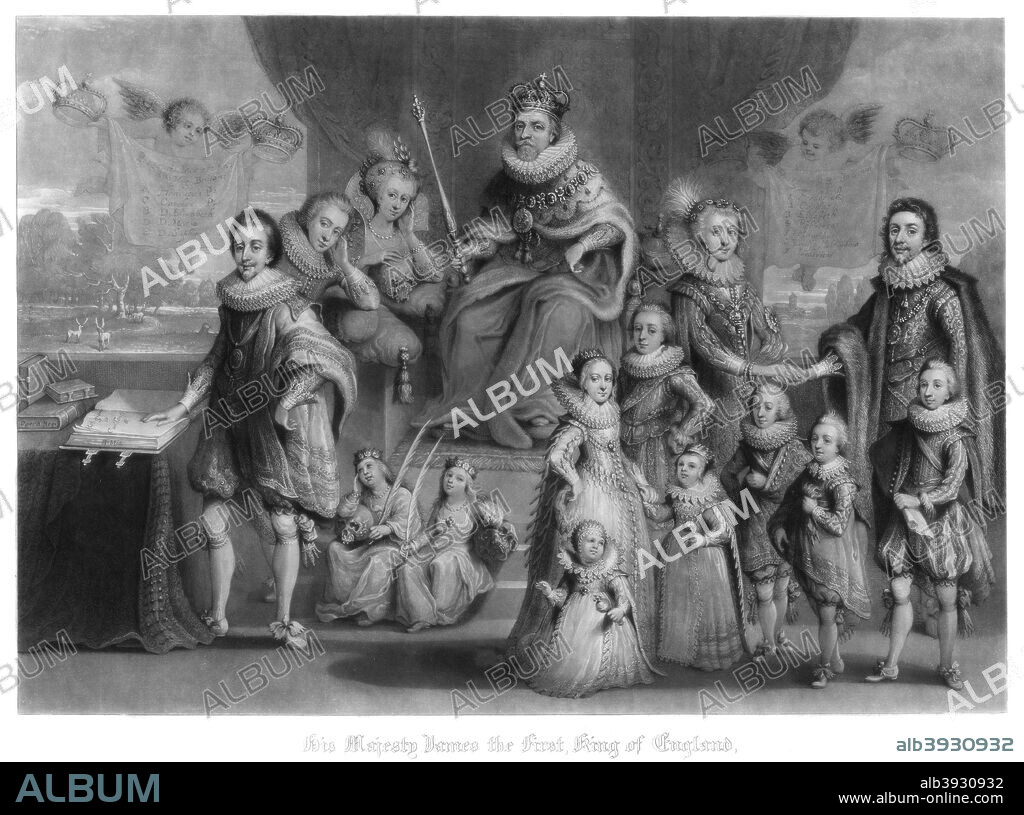The black and white drawing depicts a royal family with the king prominently seated on a throne at the center. The king is adorned in older Victorian-style royal attire, complete with a staff and an elaborate neckpiece. To his right, a woman holds a gentleman's hand, hinting at an arranged marriage within the family, surrounded by their three daughters and four sons. To the left of the king, two women lean on pillows; one may be his wife, and a gentleman stands beside them with his hand over a book, suggesting a lord or noble figure. The scene includes additional children and women, positioned intricately around the throne. The background features draped curtains, enhancing the royal ambiance. The rectangular image has a blue footer with the word "ALBUM" in all caps, and a website address and serial number in white on the lower right. At the top, old script text reads "This is his Majesty, names the first king of England," overlaying the detailed illustration.